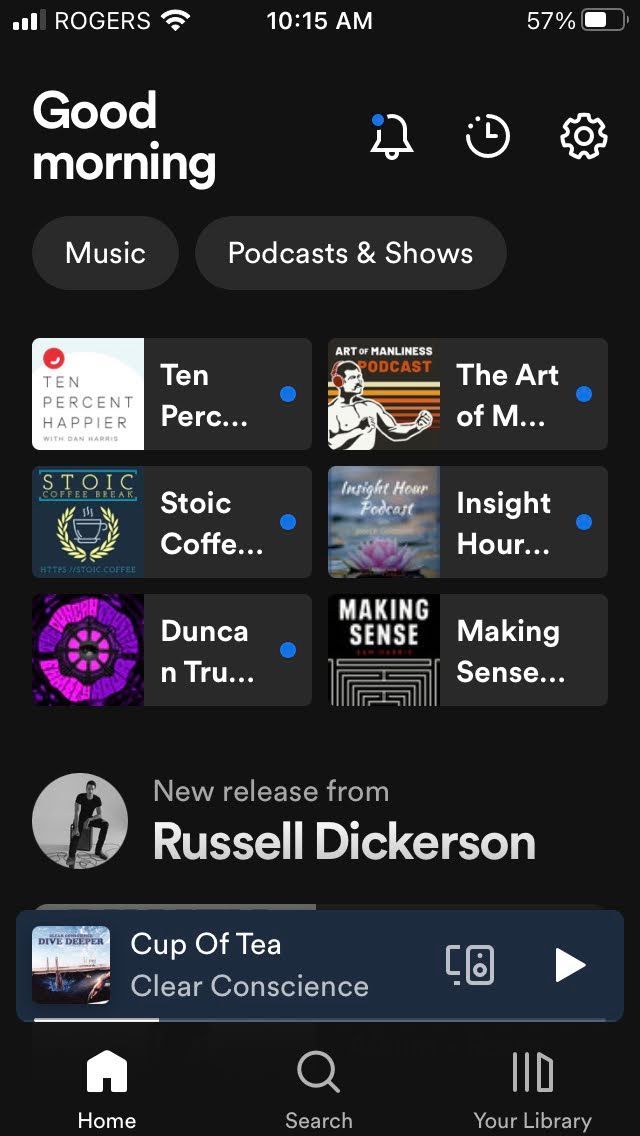This screenshot captures a smartphone interface set to dark mode. At the top of the screen, the status bar displays various icons, including the network signal icon on the left, followed by the name "Russell Rogers". Next to it, the Wi-Fi icon is visible. Centered at the top is the current time, 10:15 AM. On the right side, the battery percentage reads 57%, accompanied by the battery icon.

Beneath the status bar, a greeting message reads "Good morning," followed by categories like Music, Podcasts, and Shows. To the right of this greeting, a notification bell icon, a timer icon, and a settings icon are lined up in sequence.

Further down, the interface displays six icons representing different applications or tools: 10% Happier, Stoic, Coffee, Dunk, and Trunk, followed by "The Art of Something," and "Inside Hour." 

Additionally, there's a section highlighting new releases, specifically mentioning "New release from Russell Dickerson." The currently playing song is indicated as "Cup of Tea" by Clear Conscious.